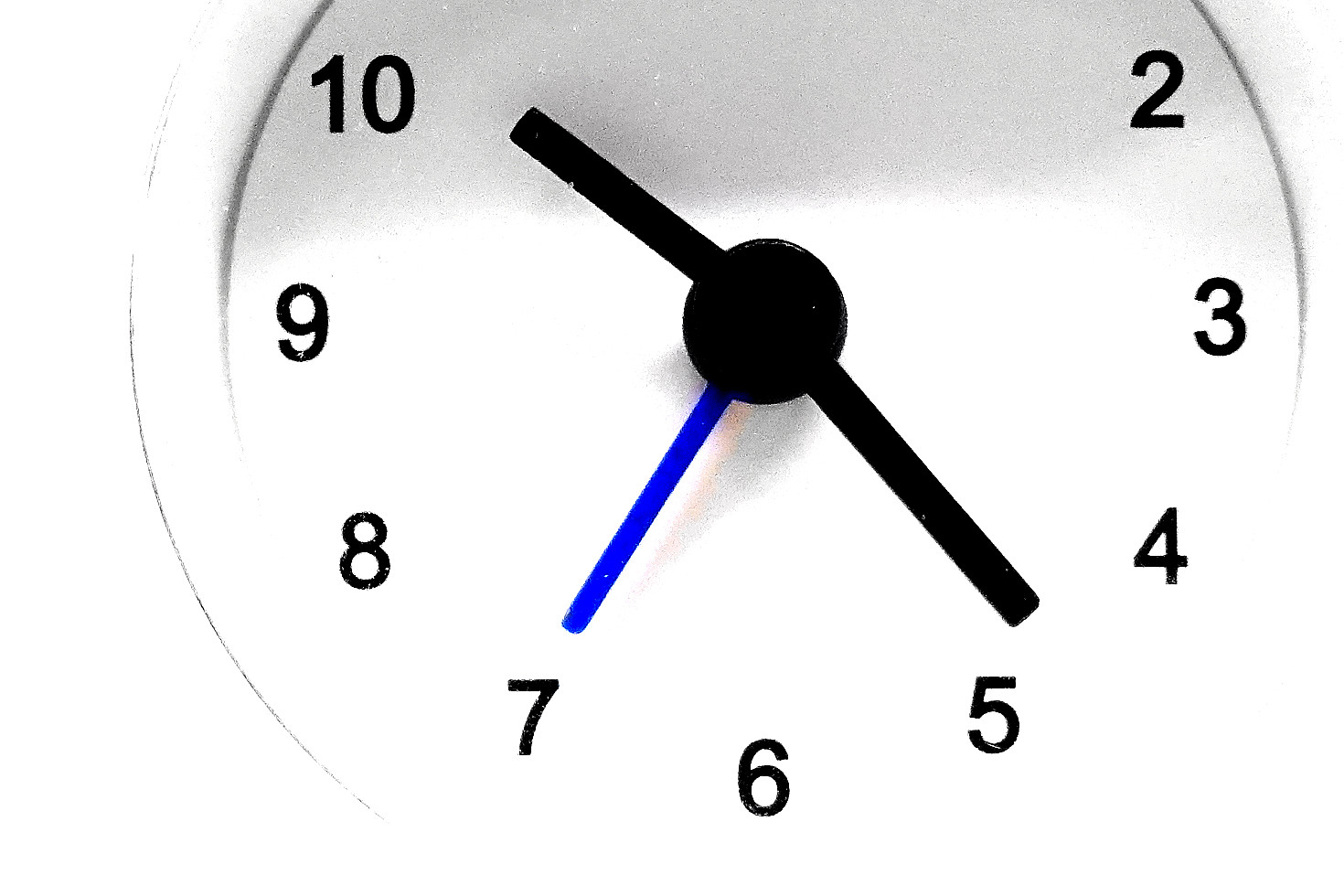This close-up image captures a round clock primarily against a white background. The clock features a white face with a partially visible white frame around it, notably cut off at the top, obscuring numbers 11, 12, and 1. The visible numbers include 10 and 2 at the top, with 3 through 10 clearly displayed along the right and bottom. The minute and hour hands are black, pointing to approximately 10:24, while the vividly blue second hand is at the 7, indicating 35 seconds. The image appears to be somewhat overexposed or faded, further blending the white clock frame into the background, and a subtle shadow is discernible near the top edge.